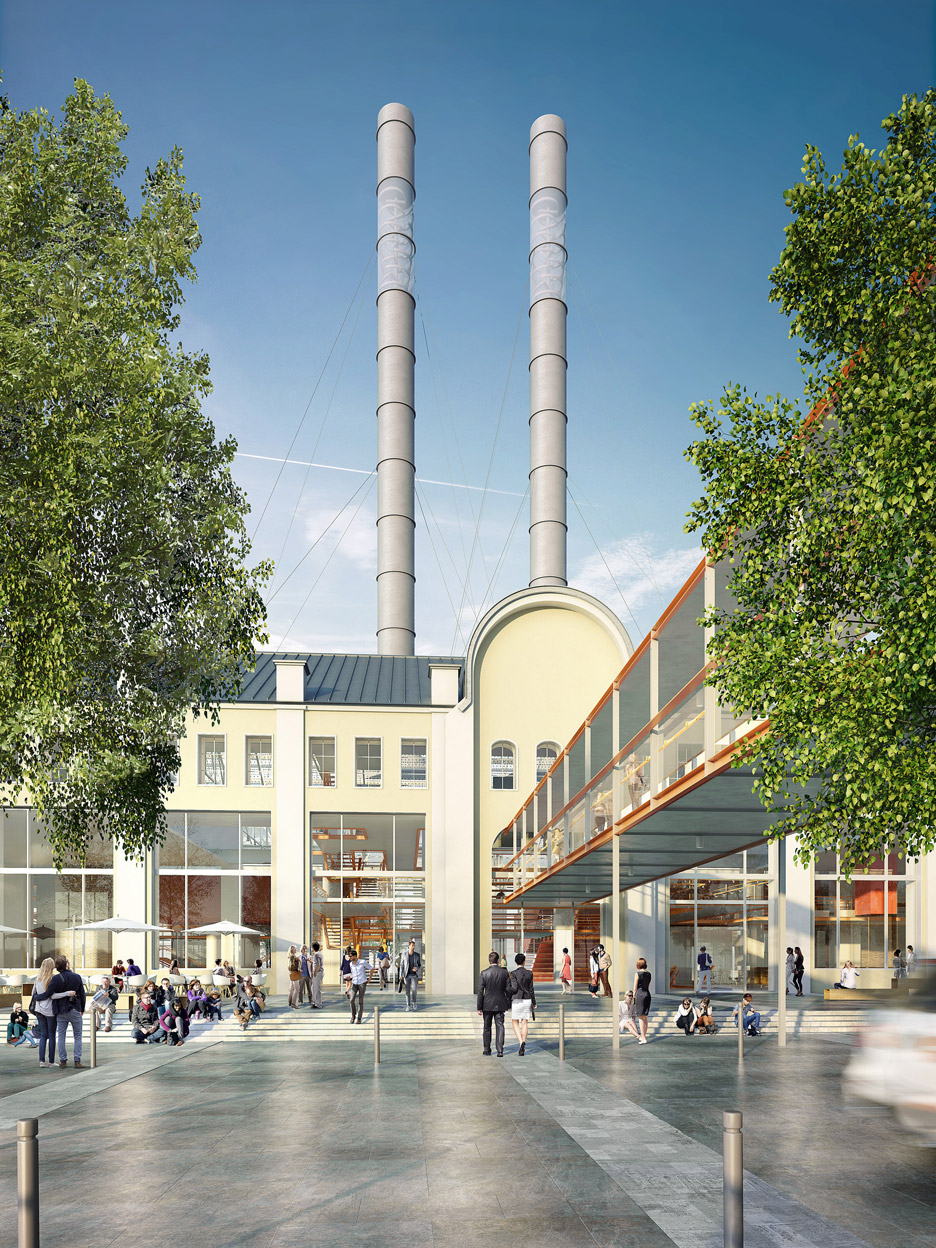The image depicts an outdoor setting showcasing what appears to be a digitally created image of a moderately tall, multi-storied building with a soft yellow facade and a blue roof. The sky above is vibrant blue with hints of scattered white clouds. The building's lower levels are dominated by large glass windows, possibly spanning the first and second stories, with a third floor featuring smaller windows. Flanking both sides of the image are green trees, their leafy canopies visible but not their trunks. In front of the building, there is a broad, dark gray sidewalk with lighter gray strips and light gray steps leading up to the entrance. The scene is bustling with people dressed in business attire, some walking up and down the steps, others leisurely seated in a designated seating area to the left, furnished with white seats and canopies. Strikingly, there are two towering, cylindrical gray stacks behind the building, supported by visible cables extending to the ground. Additionally, a prominent covered walkway extends from an upper level of the building, presumably connecting to another structure just off the right edge of the image.